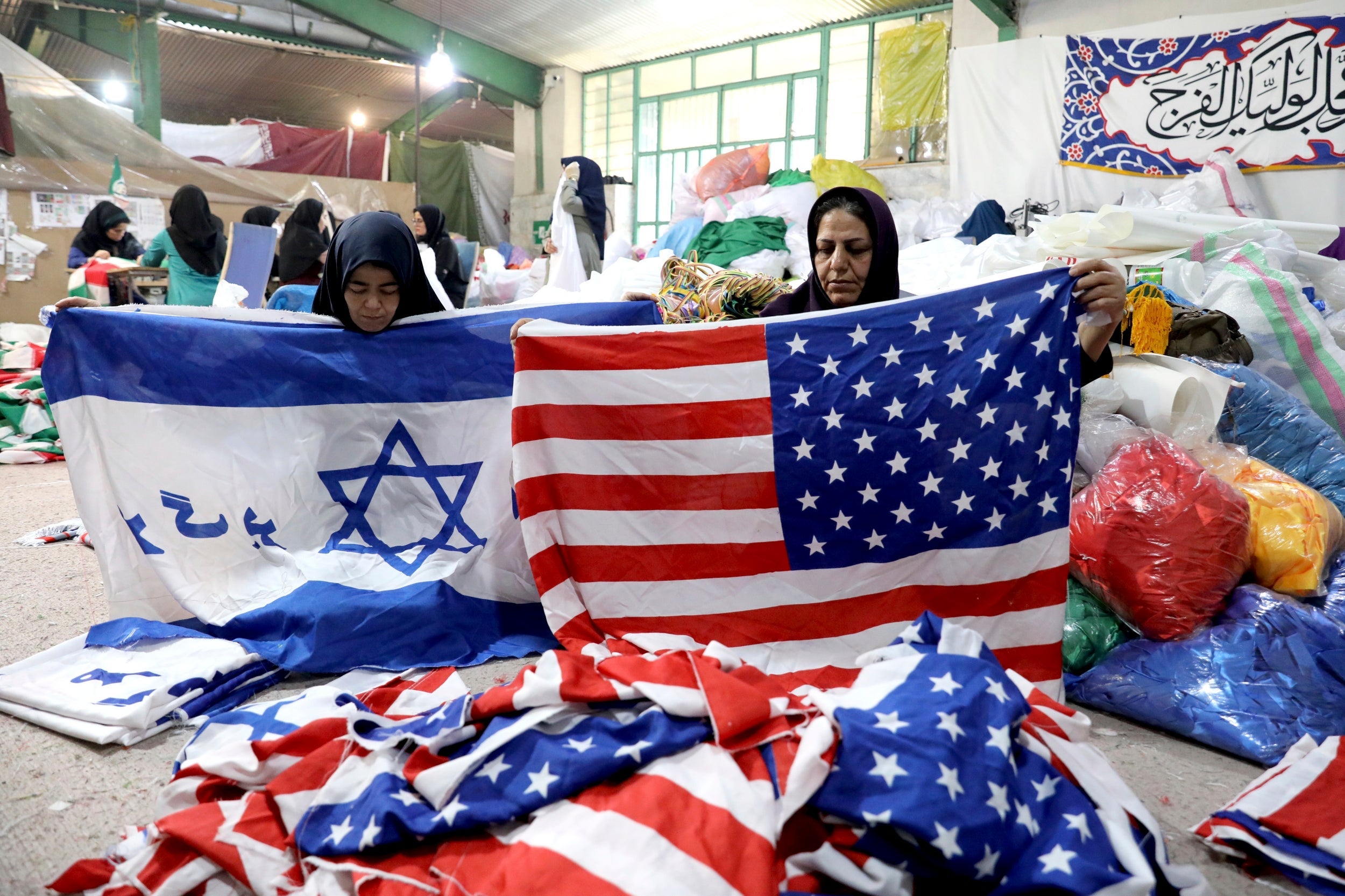The photograph captures a detailed and vibrant scene within what appears to be a warehouse setting. In the foreground, two Muslim women with head coverings are prominently featured. The woman on the right holds an American flag that is facing backwards. The woman on the left holds a blue and white flag adorned with a blue Star of David, signifying the Israeli flag. Both women are surrounded by a pile of American flags. To their right are clear plastic bags filled with colorful fabric materials, including red, blue, and yellow. 

In the background, a group of about five or six Muslim women are seated at a table, busily working on making flags. On the wall behind them hangs a banner with Arabic writing, adding cultural context to the scene. The setting, similar to a warehouse, has a mix of materials and fabric scattered around, with light suggesting it is daytime. The detailed interactions and activities of the women reveal a collaborative effort in sorting and handling fabric flags.